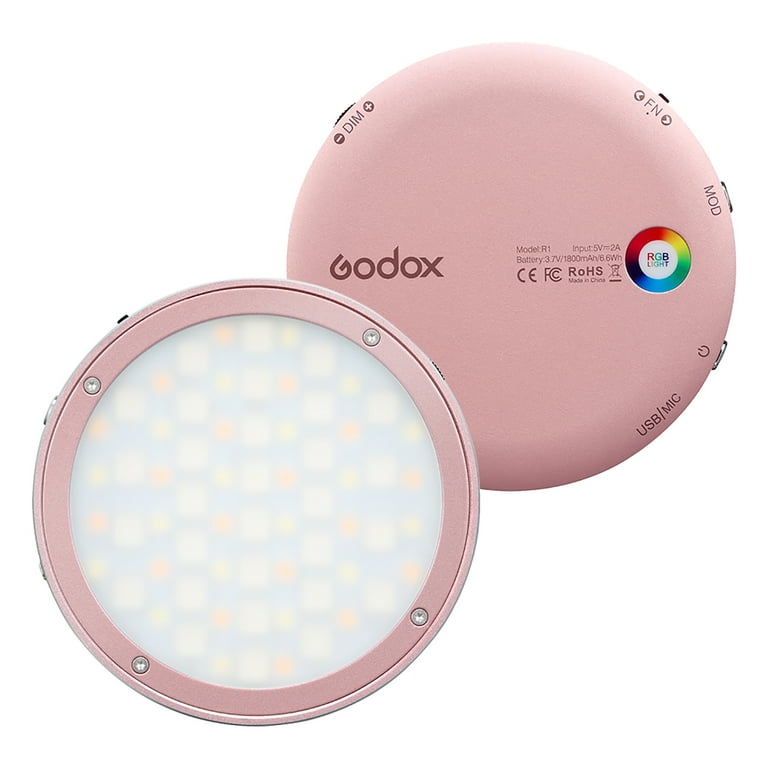This image depicts a pink electronic device, likely an LED light from "GODOX," specifically model R1. Featured are two views: the front and the back. The front is dominated by a large screen, while the back sports a more detailed interface. Central to the back is a color wheel with "RGB Light" inscribed. Surrounding it are several controls: a "DIM" button with plus and minus symbols, an "FN" button flanked by left and right arrows, a "MOD" button, and a power switch. Additionally, there's a slot labeled "USB/MIC." The pink outer casing is secured by four screws and has numerous printed details, including the power specifications (Input: 5V=2A; Battery: 0.37V/18 mAh/6.6 WH) and compliance marks (CE, FC, ROHS).